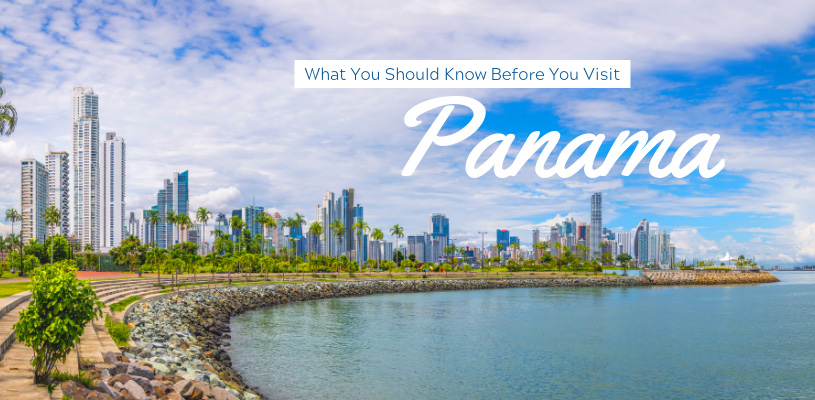This postcard from Panama Beach features a captivating view that blends natural beauty with urban charm. The top two-thirds of the image is dominated by a vibrant sky, with shades of blue in the upper left corner gradually transitioning to areas covered by fluffy white clouds. The sky meets the city skyline, which is beautifully captured just right of center. 

In the middle of the postcard, a bold white rectangle prominently displays text in blue letters that reads, "What You Should Know Before You Visit." Below this, in cursive white lettering, the word "Panama" is elegantly written.

Moving down from the skyline on the right side, around an inch in and extending downward and slightly leftward to about two-thirds of the image, the scene transitions into a serene expanse of blue water. Along the edge, mingling with the water, is a stretch of sandy shore mixed with rocks.

Below the sky, the city skyline stands tall, punctuated by a striking palm tree leaf that extends above the buildings on the left side. Bushes and palm trees line up in front of the buildings, creating a lush barrier that stretches across the scene. A small patch of grass is visible in front of the palm trees.

On the left side of the image, a little walkway can be seen, extending upwards and to the right for about two inches. At the bottom of the postcard, approximately an inch from the left edge, a well-maintained bush is situated. In front of this bush, a thin strip of grass runs upward and to the right, adding a final touch of green to this picturesque coastal view.